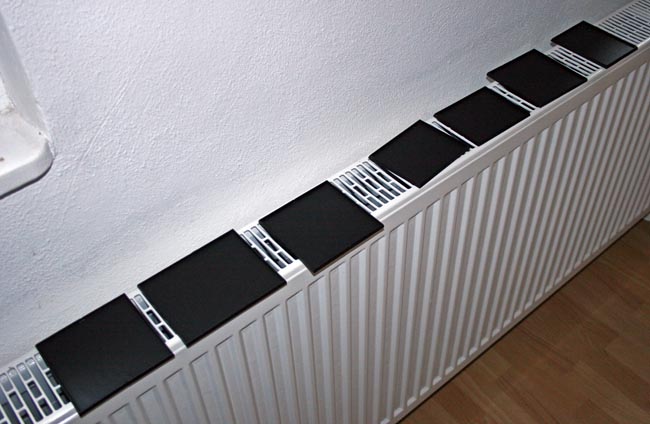The image depicts a white radiator against a textured white wall, resembling popcorn ceiling texture but on a vertical surface. The radiator features vertical slats leading down to a light-colored hardwood floor, bordered by a white baseboard. A white windowsill sits above the radiator, suggesting the presence of a window. The radiator has a protective grate on top, displaying seven evenly spaced black rectangles or squares, possibly made of ceramic material. These black patches, which irregularly dot the radiator's surface, might be there to dry out or to serve as small shelves that could hold knick-knacks or plants, thus preventing direct contact with the heat. The wall shows signs of imperfection, with bubbles in the paint and grayish areas disrupting its otherwise white appearance.